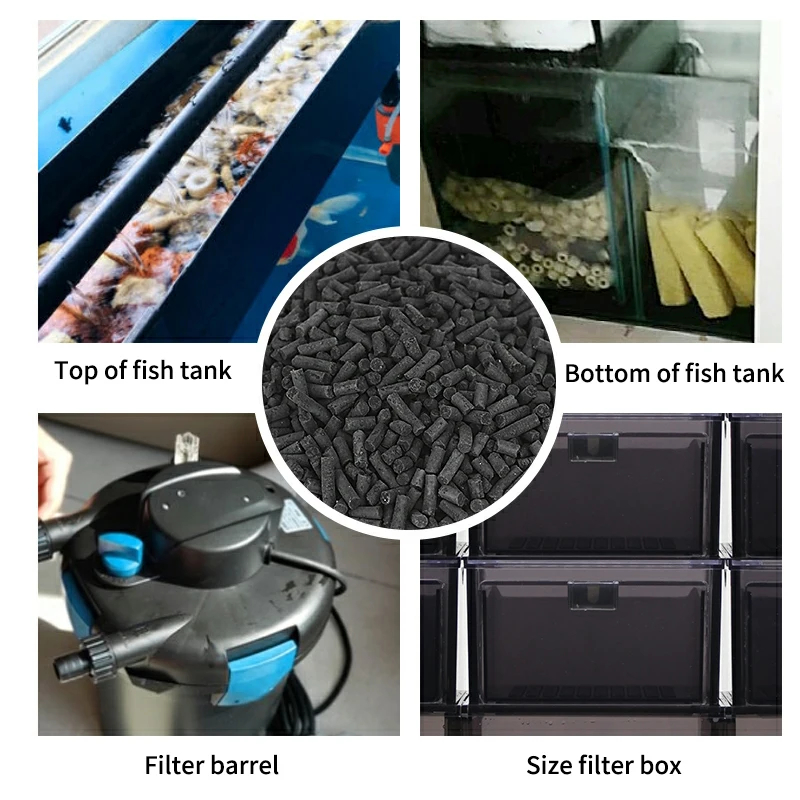This promotional brochure for an aquarium filter system is composed of four square images surrounding a central circular image. The circular image in the center displays black cylindrical pellets, likely charcoal filter pieces used for purifying water. The top left image, labeled "Top of Fish Tank," offers a view looking down into a fish tank, showcasing clear water, some coral, and possibly a koi fish. The top right image, labeled "Bottom of Fish Tank," reveals the tank's base, featuring a pane of glass and several yellowish circular items. The bottom left image, labeled "Filter Barrel," depicts a plastic filtration device and a portion of a man's hand, illustrating how water is pumped and purified through the barrel. The bottom right image, labeled "Size Filter Box," shows containers designed to hold replacement filters essential for maintaining the filtering system. Together, these images highlight the components and functionality of the aquarium filter system.